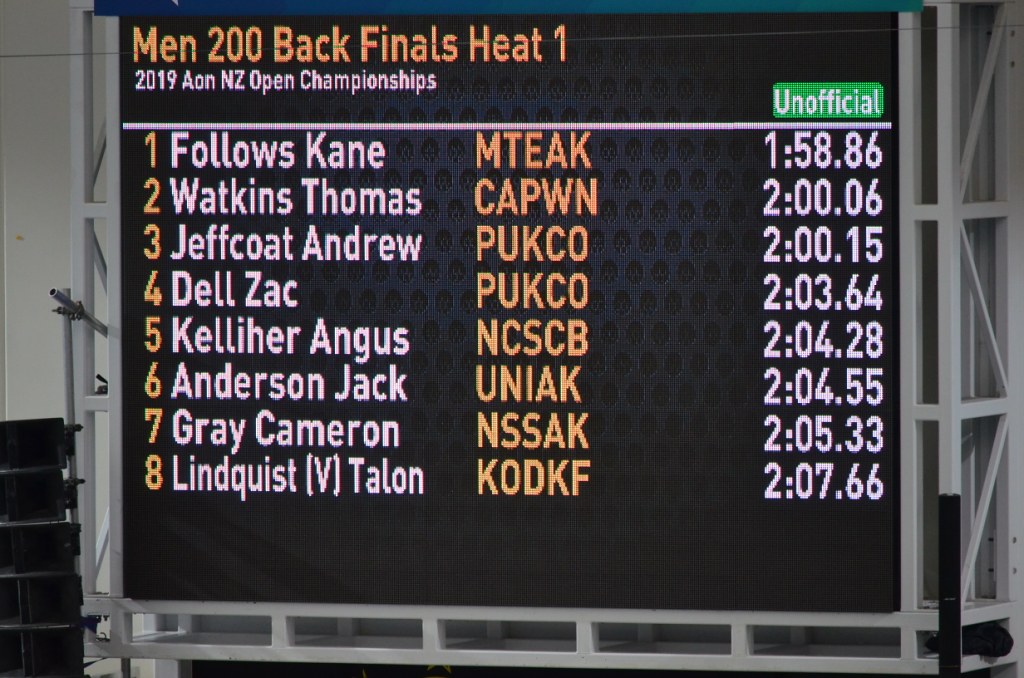The image showcases a black, square scoreboard mounted on a silver metal frame. This scoreboard details the "Men 200 Back Finals Heat 1" at the "2019 AON NZ Open Championships" in bright orange and white lettering. It displays the names of eight athletes along with their unofficial times. From lanes one to eight, the athletes listed are Follows Kane, Watkins Thomas, Jeffcoat Andrew, Delzak, Kelleher Angus, Anderson Jack, Gray Cameron, and Lindquist V. Tellen. The left side of the scoreboard enumerates their respective lanes, while the right side shows their recorded times, providing a comprehensive view of the competition's results.